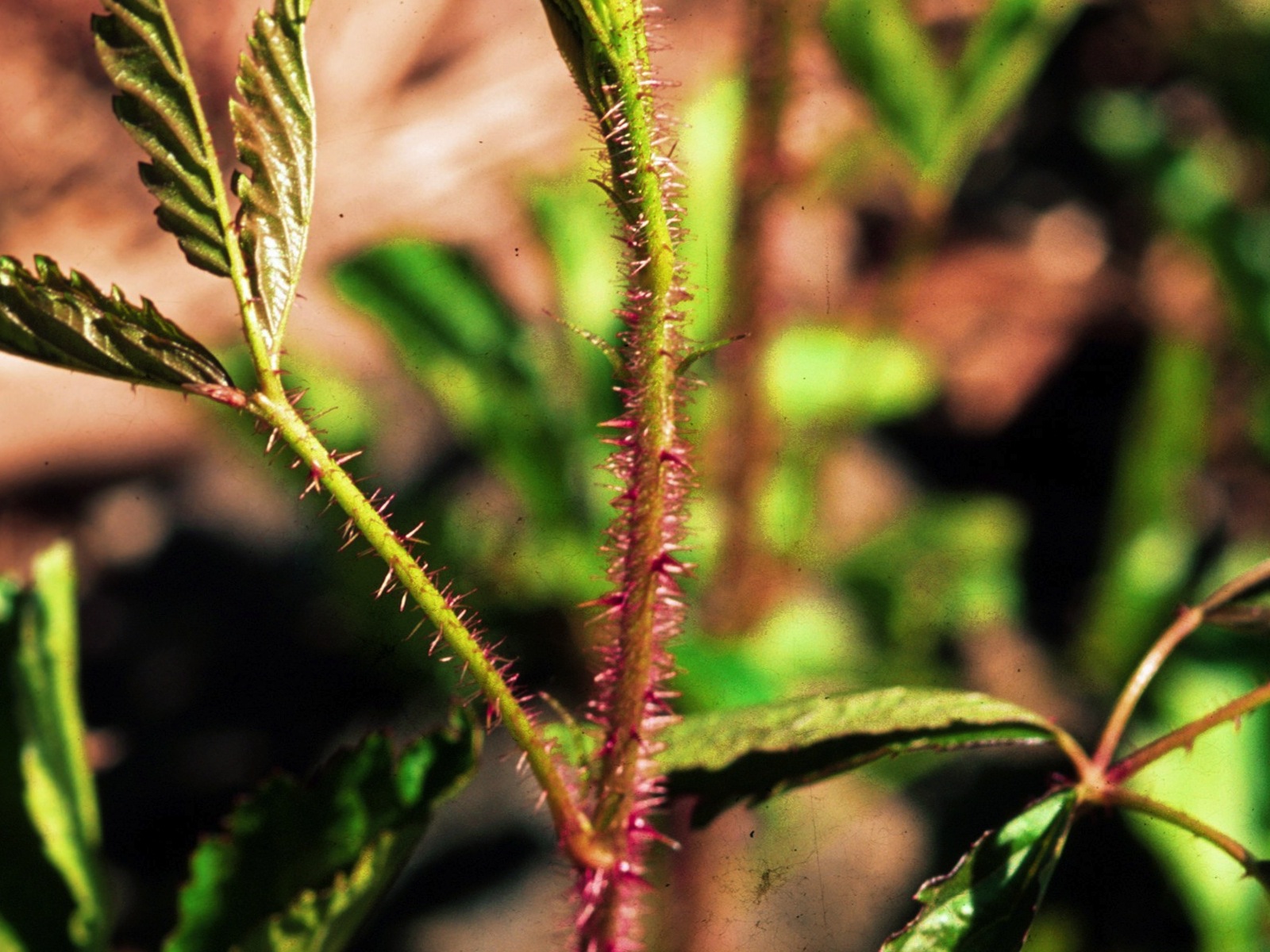This close-up photograph captures the vivid details of a unique plant in a forest setting. The primary focus is on a long green stem that transitions to brown towards the base, densely covered with pink prickly thorns, particularly abundant along the central stem. To the left, another vibrant green stem with leaves at the tips stands out, also adorned with similar pink thorns. The background is a blur of greenery and earthy browns, suggesting a lush forest environment, with light reflected off possible rocks or tree trunks, adding subtle highlights of green and brown hues. Shadows play across the scene, further enhancing the depth and focus on the striking plant structure in the foreground.